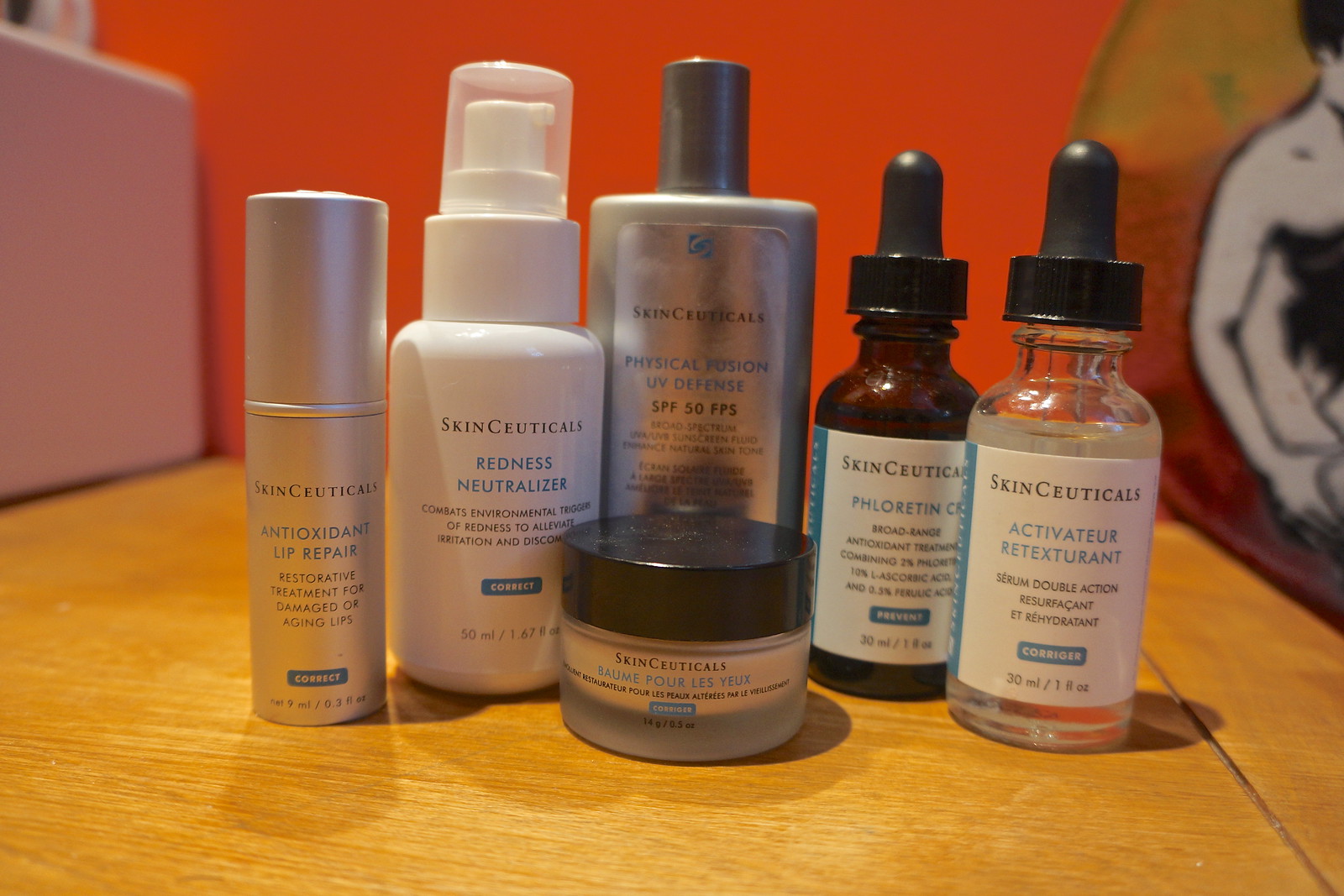In this image, a wooden table or countertop serves as the base for a carefully arranged selection of toiletries. Central to the arrangement is a collection of bottles, five in total, spanning from left to right. Notably, two of these bottles on the right are equipped with droppers. The middle item is distinctively shorter and rounder compared to the others. 

Detailing the items from left to right: the first bottle is white and comes with a spray nozzle; the second bottle, positioned in the middle, has a black lid and bears the label "Antioxidant Lip Repair"; next to it, a cylindrical silver bottle marked "Redness Neutralizer"; followed by a product labeled "SPF 50"; and finally, another product from the brand SkinCeuticals, with some text potentially in French that’s not fully legible in the image.

The background features an orange wall, adding warmth to the scene. To the left, there's a pink box, while to the right is what appears to be an artwork depicting a man. This background is slightly blurred, making it challenging to discern finer details. 

The overall composition brings a vibrant and eclectic mix to an otherwise everyday scene, capturing the essence of a personal care space.